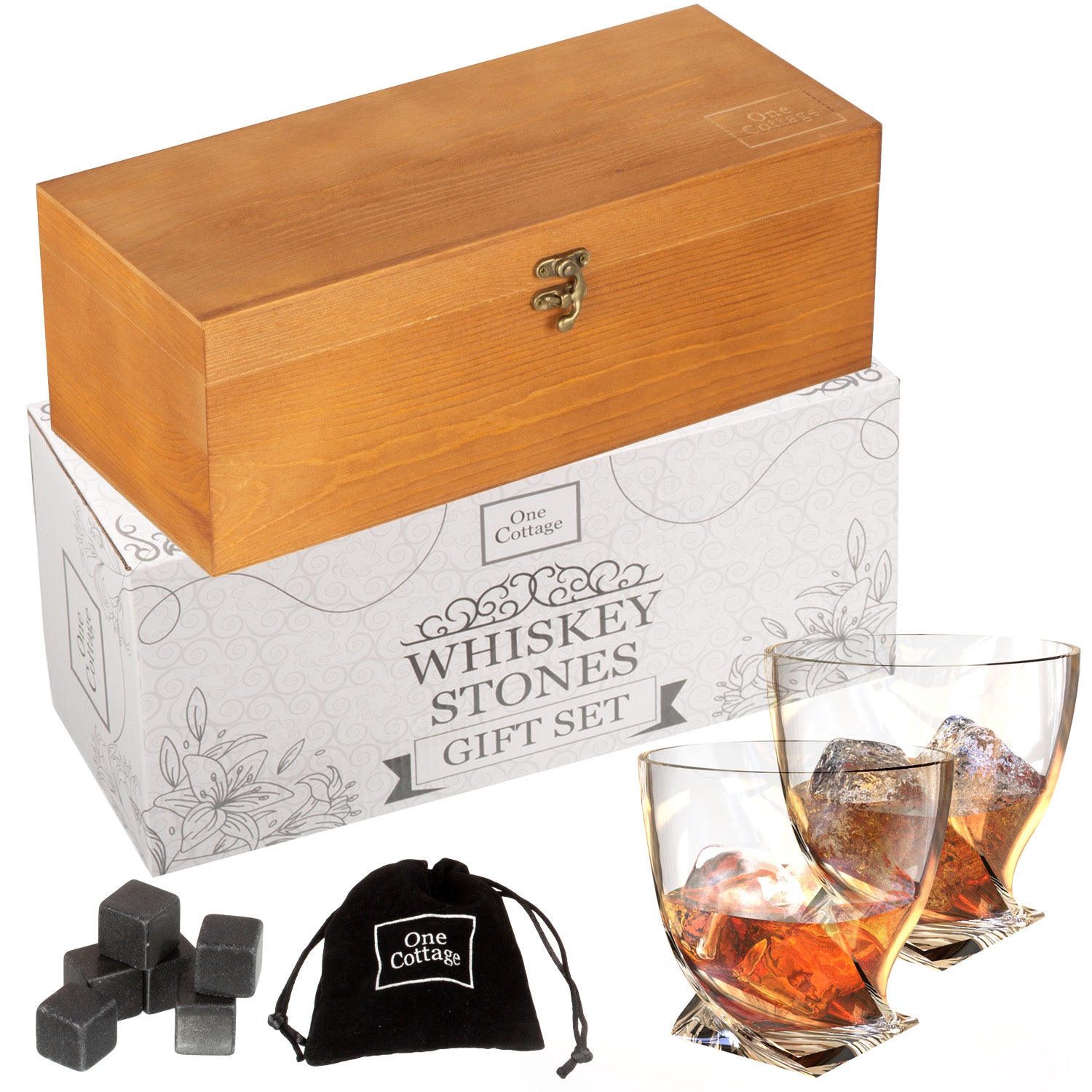The image showcases an elegant whiskey gift set. At the top center, there's a light brown wooden box with a silver latch in the front. This box is slightly angled down to the left and its lid is open. Beneath this wooden box, there's a refined white box adorned with floral and swirly gray patterns on its bottom corners. In the center, the white box features a black square with the words "One Cottage" inscribed inside. Below it, "Whiskey Stones" is boldly written in black lettering, followed by a white banner proclaiming "Gift Set" in black text. 

Arranged in front of the box, starting from the left, are six small gray cubes resembling ice cubes. To their right is a black drawstring pouch bag, featuring a white square with "One Cottage" printed in the center. Further to the right, there are two unique glasses each filled halfway with an amber liquid, presumably whiskey, containing visible ice cubes. The glasses have a distinctive twist design as they rise halfway from their flat base to their normal rim.